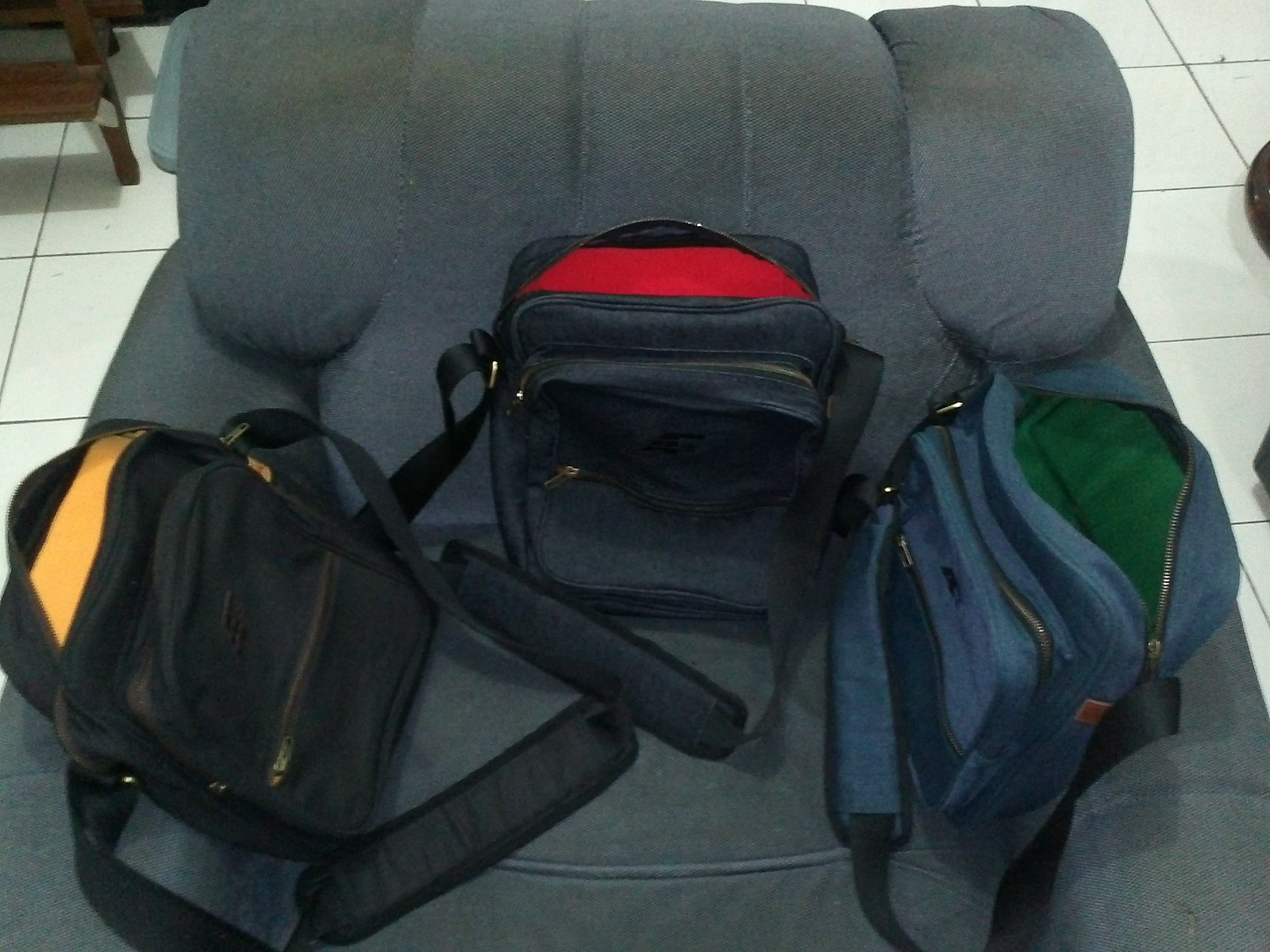This detailed photograph captures a scene centered around an old, dark blue and gray worn-out chair with dirty and heavily used cushions. The chair, likely situated in a kitchen judging by the background, is resting on a white tiled floor with black lines. On the top left corner of the image, part of a black stool is barely visible, while small black circles appear to intrude from the right side of the frame.

On this dilapidated chair are three fabric pouch-like bags, resembling lunch coolers, each distinct yet sharing some similarities. The bag on the left is a blackish color with an open zipper revealing a yellow interior compartment and a strap for carrying. The middle bag has a navy exterior with its zipper also open, showcasing a deep red inside and a laying handle at the front. Lastly, the bag on the right is a lighter navy blue and its unzipped compartment reveals a hunter green interior. All three bags feature multiple zipper sections, including a larger section, a smaller section, and a front pocket, with shoulder straps designed for easy carrying.